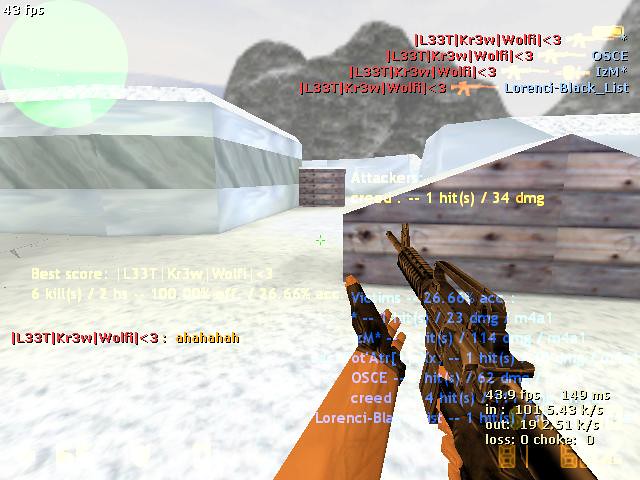The image is a high-resolution screenshot from a first-person shooting video game set in a snowy landscape. The player's perspective shows them holding a gun with their right hand, while their gloved left hand is poised to grab the barrel. The environment features diverse elements including a large white tent with a gray stripe, a small angled wooden building on the right, a big wooden crate in the back left, a significant snow drift, and jagged rocks in the background.

The game's Heads-Up Display (HUD) is filled with information. At the top left corner, the FPS (frames per second) is displayed. The top right corner details the team's available weapons. In the center-right, it shows "Attackers" along with the damage stats (e.g., "attacks 1, hits 34 DMGs"). Directly in the middle, a line of text lists the top player's score, including details like "43FPC, best score: L33T KR3W WOLF, six kills." The bottom right corner shows the player’s individual stats in light blue, which is somewhat hard to read. The immersive design of the game captures the intense, war-like atmosphere through its detailed overlay and environment.